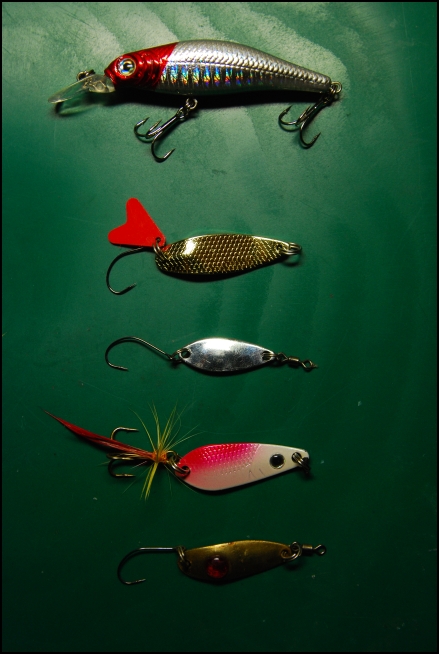The image is a color photograph of an assortment of fishing lures displayed against a dark green, textured background with some scratches and specks. The backdrop is not smooth and becomes lighter towards the top due to a light source.

At the top of the image is a lure designed to resemble a small fish. It has an iridescent white or silver body with a red head, complete with an eye that has a black pupil. This lure is detailed with multiple hooks: one at the back and one in the middle.

Beneath the top lure is another featuring a red, heart-shaped component, along with hooks positioned on it. 

Below this is a silver, flat lure shaped like an oval, with a single hook on one end and a metallic piece at the other.

The next lure down has a combination of white and pink coloring and features a feather-like tail with green strings and a red extension. It has hooks positioned on both ends.

At the bottom of the image, there is a small gold lure with a black hook at the rear and what appears to be a bead on its front center. 

Altogether, the array of lures vividly showcases a variety of colors, shapes, and intricate details designed to attract fish.